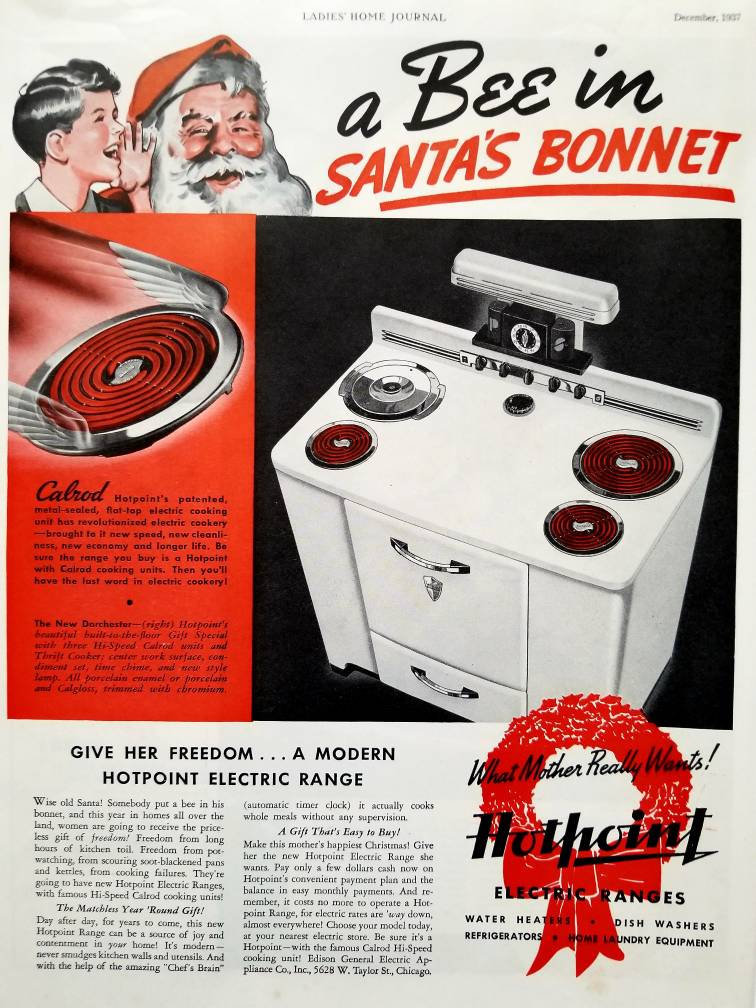In the December 1937 issue of Ladies' Home Journal, there is a detailed full-page advertisement for a Hotpoint electric range. The ad, titled "A Bee in Santa's Bonnet" in large letters with "Santa's Bonnet" underlined in red, features an illustration of a young boy with black hair whispering into the ear of a smiling Santa Claus at the top left corner. The background text indicates it's a holiday-themed ad, appealing to Christmas gift-giving sensibilities.

On the right side of the page, there's a full image of the advertised Hotpoint electric range, showcasing its sleek, white design with black, spiraled stovetop burners. The stove features four burners, two large at the back and two smaller at the front, with a notable large space in between them and a metal cover over the back left burner. The stove also includes various advanced features such as drawers underneath, a little dial clock on the front, and other modern conveniences for that era.

Additional visual elements include a red wreath with a bow in the bottom right corner, enclosing text that reads "What Mother Really Wants," followed by "Hotpoint Electric Ranges, Water Heaters and Dishwashers, Refrigerators, and Home Laundry Equipment." Central to the ad's promotion, the range boasts Hotpoint's patented "Calrod" cooking units, which promise improved speed, cleanliness, economy, and durability. Descriptive text highlights the range's modern attributes such as "three high-speed Calrod units, thrift cooker, center work surface, condiment set, time chime, and new style lamp," all trimmed with chromium and finished in porcelain enamel.

The slogan at the bottom of the ad encapsulates the product's selling point: "Give Her Freedom, a modern Hotpoint electric range," emphasizing the liberation and convenience the new technology brings to household cooking.